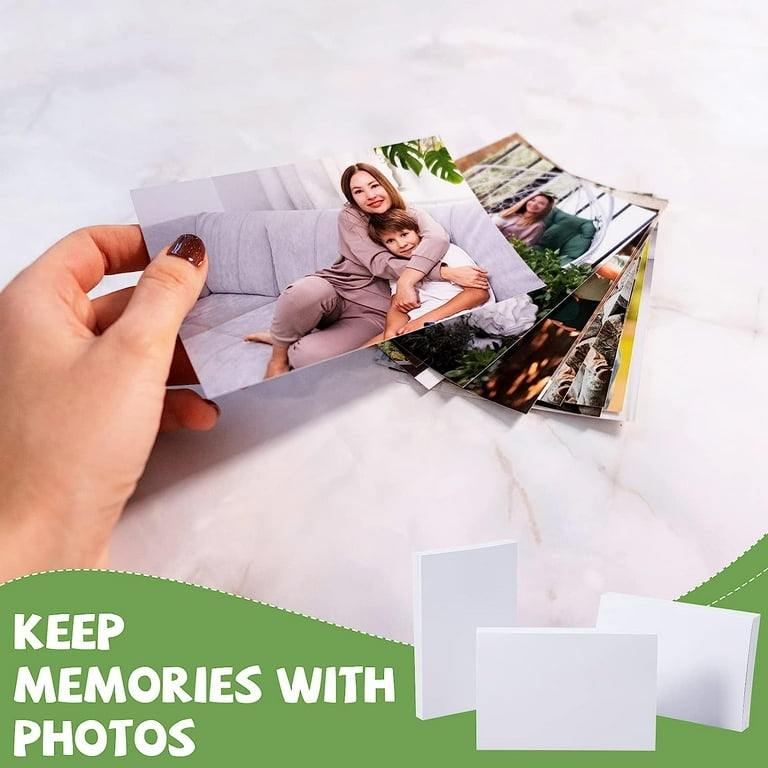This rectangular advertisement, slightly taller than wide, features a combination of images and text promoting photo printing. The backdrop is a cream-colored background with white marble, overlaid with a green, wave-shaped border at the bottom. In bold white block letters, it reads "Keep memories with photos." To the right of this text are three blank photo canvases or stacks of photo paper, shaped like index cards. 

In the foreground, a woman's left hand, with dark red nails speckled with gold, holds a stack of photographs. The top photo shows a woman in a maroon-pink pajama set hugging a small boy in a white t-shirt as they sit on a couch adorned with houseplants in the background. The woman has long hair, is barefoot, and wears pink lipstick, while the boy appears somewhat unhappy. Behind this photograph, another picture shows the same woman sitting on an outdoor chair surrounded by more houseplants. The remaining photos are indiscernible. This advertisement emphasizes preserving cherished moments through printed photos, blending a homely and nostalgic atmosphere.